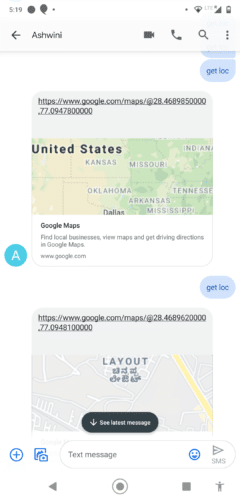A blurry and small screenshot of a phone app interface displays an attempt to find website results on Google. At the top of the screen, there is a back arrow followed by the name "Ashwini." On the right-hand side, there are icons for video, phone, search (magnifying glass), and a vertical ellipsis. The screen is not a chatbot interface as indicated by several blue boxes. One blue box says "Get location," followed by a URL: "https://www.google.com/maps/". The user's location is indicated as the United States, focusing on Missouri and the Oklahoma panhandle area. The screen shows Google Maps with features to find local businesses, view maps, and get driving directions. A small blue circle with a red 'A' is present, suggesting an interactive element, possibly a chatbot. There's another mention of "Get location," and a more zoomed-in view reveals text in Chinese characters on a map. At the bottom center, a black button reads "Save Later" with a down arrow. Below this, a box labeled "Text message" is visible, likely indicating an option for messaging.